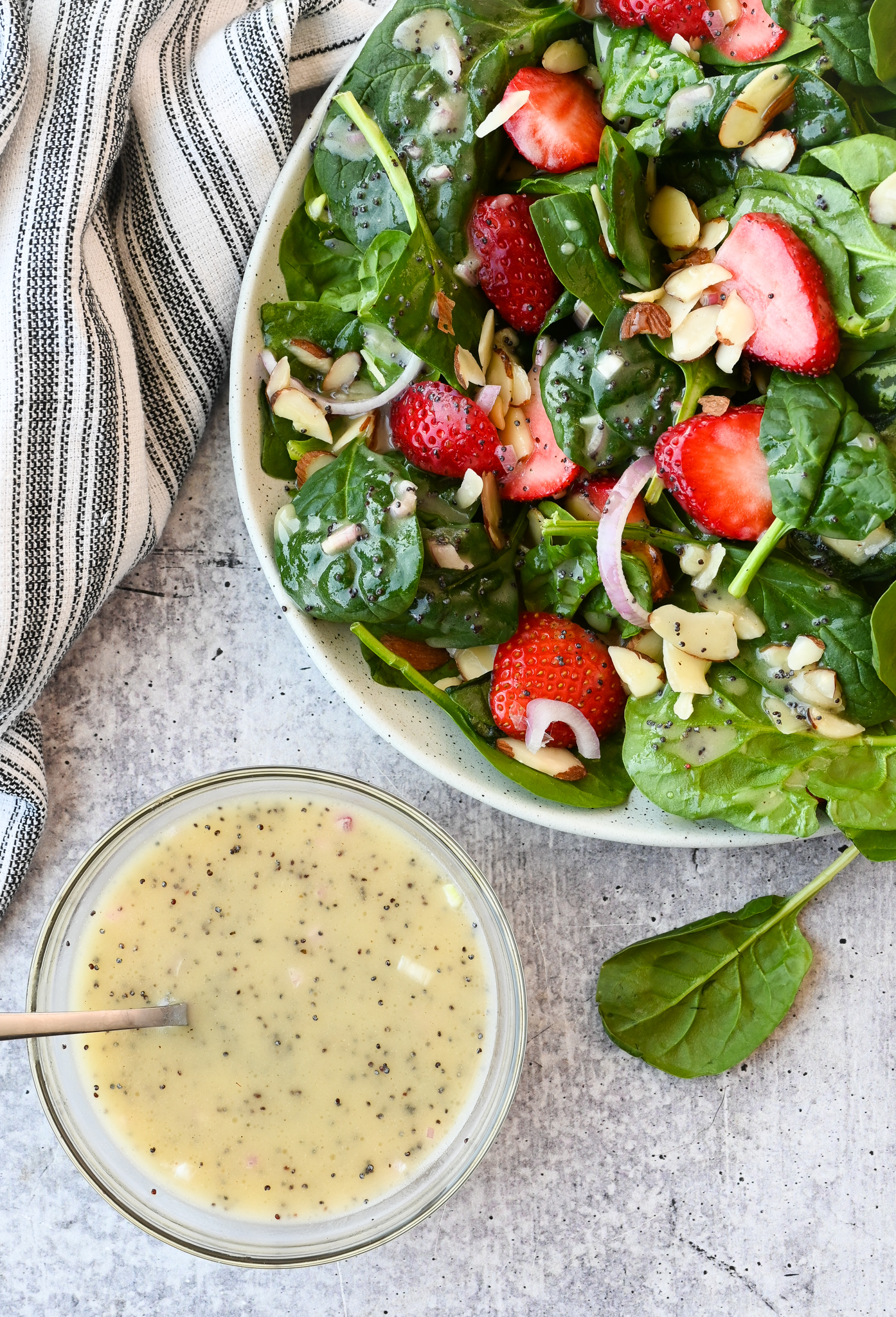The image depicts a detailed overhead view of a white-painted, grayish-white tabletop featuring two distinct bowls. In the upper right-hand part of the photo, a large white bowl brims with a vibrant salad composed of lush green spinach leaves, halved strawberries, sliced purple onion rings, and chopped nuts, likely almonds. This bowl is partially resting on a slightly scrunched, black and white striped linen napkin located in the upper left corner of the image. To the lower left-hand corner, a smaller, clear bowl with a bronze rim and a shiny silver-golden spoon contains a yellow, creamy vinaigrette dotted with black specks, likely pepper. Some of the dressing has already been drizzled over the salad, adding a glistening finish to the fresh ingredients. A single spinach leaf has fallen outside the white bowl, enhancing the natural and inviting presentation of the meal.